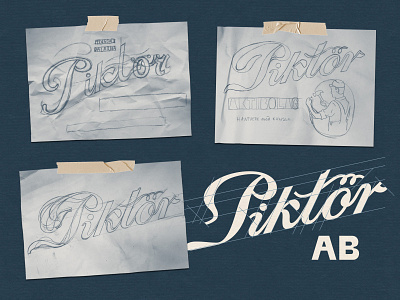The image showcases a dark blue background with three gray sketches taped onto it. These sketches depict the word "PIKTOR" in various stylized letterings. In the upper right corner, in white text, it reads "PIKTOR A-B." One of the sketches features a detailed drawing of a man, possibly a carpenter, wearing a hat and overalls, hammering a nail. This particular sketch emphasizes the craftsmanship theme related to the name PIKTOR. The sketches are intricately taped to the dark blue background, forming an artistic layout reminiscent of an advertisement.